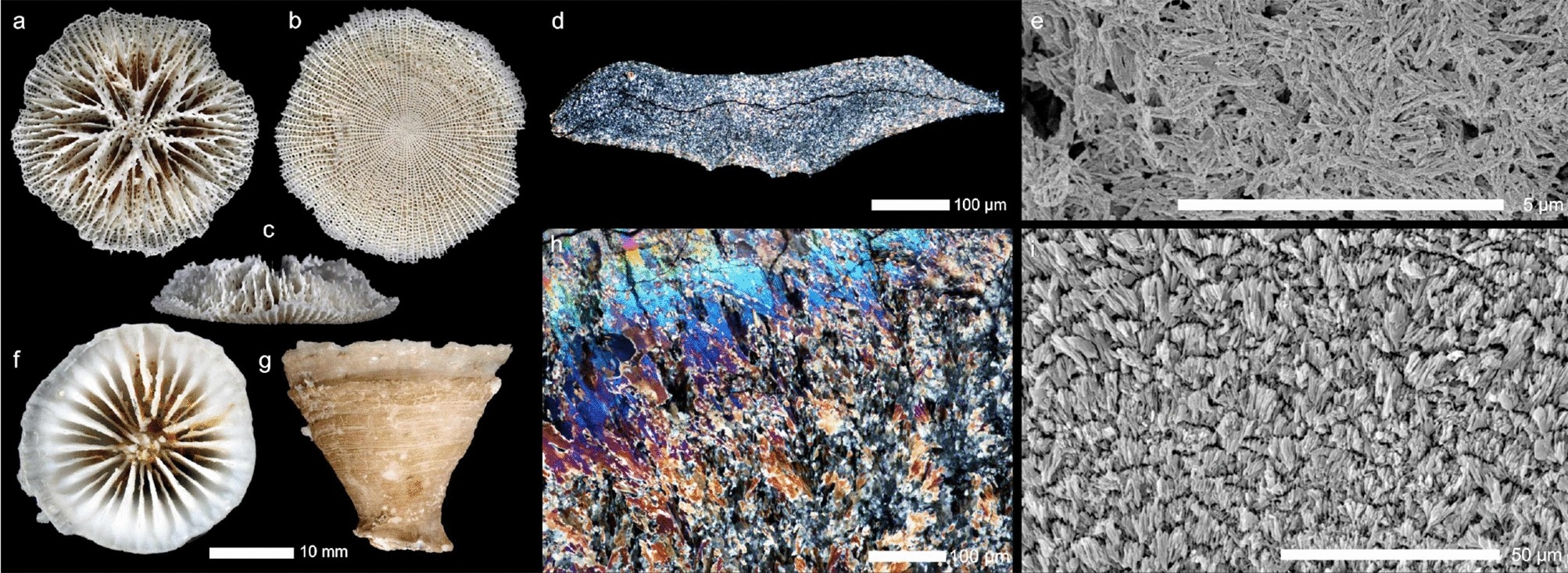This detailed close-up image, potentially a microscopic view of various specimens, features a black background with nine labeled objects arranged in an intricate pattern. Each object is marked with a letter from A to I. In the top row, from left to right, are A, B, D, and E. Below and between A and B is C, which stacks vertically with F and G. To the right of G are H and I.

- **A:** A circular specimen resembling a shell with numerous holes, evoking a porous coral structure.
- **B:** Another circular, shell-like specimen next to A, appearing sandier with fewer holes.
- **C:** Situated below A and B, this specimen, viewed from the side, has a spiky, irregular texture, possibly another type of shell.
- **D:** A horizontally elongated piece of black rock, distinct in its simplicity compared to the more detailed specimens around it.
- **E:** A highly magnified close-up showing a labyrinth of gray lines and shapes, perhaps depicting the intricate internal structure of a rock.
- **F:** Below C, similar in pattern to A but with white stripes and a more defined border.
- **G:** Adjacent to F, a seashell-like object with a brownish hue, likely viewed from the top.
- **H:** Displaying a vibrant rock with multicolored elements, reminiscent of an oil spill's iridescence.
- **I:** Similar in its gray-toned complexity to E, but with a denser packing of lines and forms.

This arrangement suggests a study or diagram of marine life or geological specimens, captured in various angles and magnifications to showcase their diverse textures and structures.